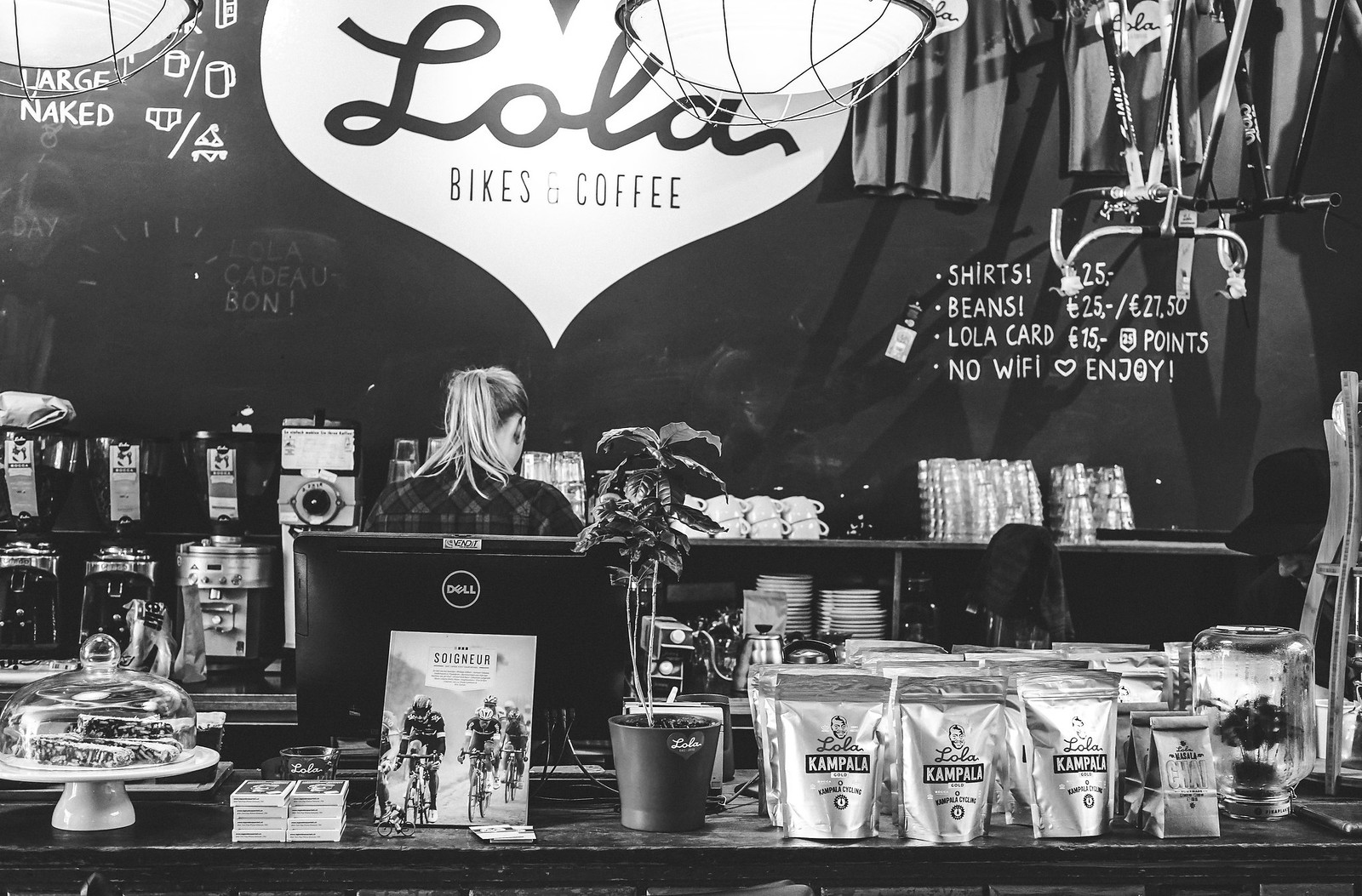This black-and-white photo captures the interior of a bike-themed coffee shop named Lola Bikes and Coffee. Dominating the center of the back wall is a large, white heart logo with "Lola" written in black cursive, and beneath it, the words "Bikes and Coffee." To the right of the heart, there are handwritten signs in white, listing items such as shirts ($25), beans ($25), and the Lola card ($15), along with the phrases "No Wi-Fi," "Heart," and "Joy." The signs have a charming, artisanal touch.

In the foreground, a Dell computer monitor is prominently positioned in the center of the counter, partially obscured by a potted plant. To the right of the monitor, there are various types of coffee, including bags labeled "Lola Compala," perfect for take-and-go customers. On the left side of the counter, there is a covered platter, potentially filled with pies or other desserts.

A barista, wearing a plaid shirt with her back to the camera, is working behind the counter. She is stationed near an array of coffee machines on her left. The setting is warm and inviting, exuding a sense of community and craftsmanship. To the extreme right, partial writings suggest options for different coffee servings, possibly labeled "large" and "naked," alongside small drawings. The ambiance is completed with an advertising sign featuring bicyclists, echoing the shop's bike-friendly theme.